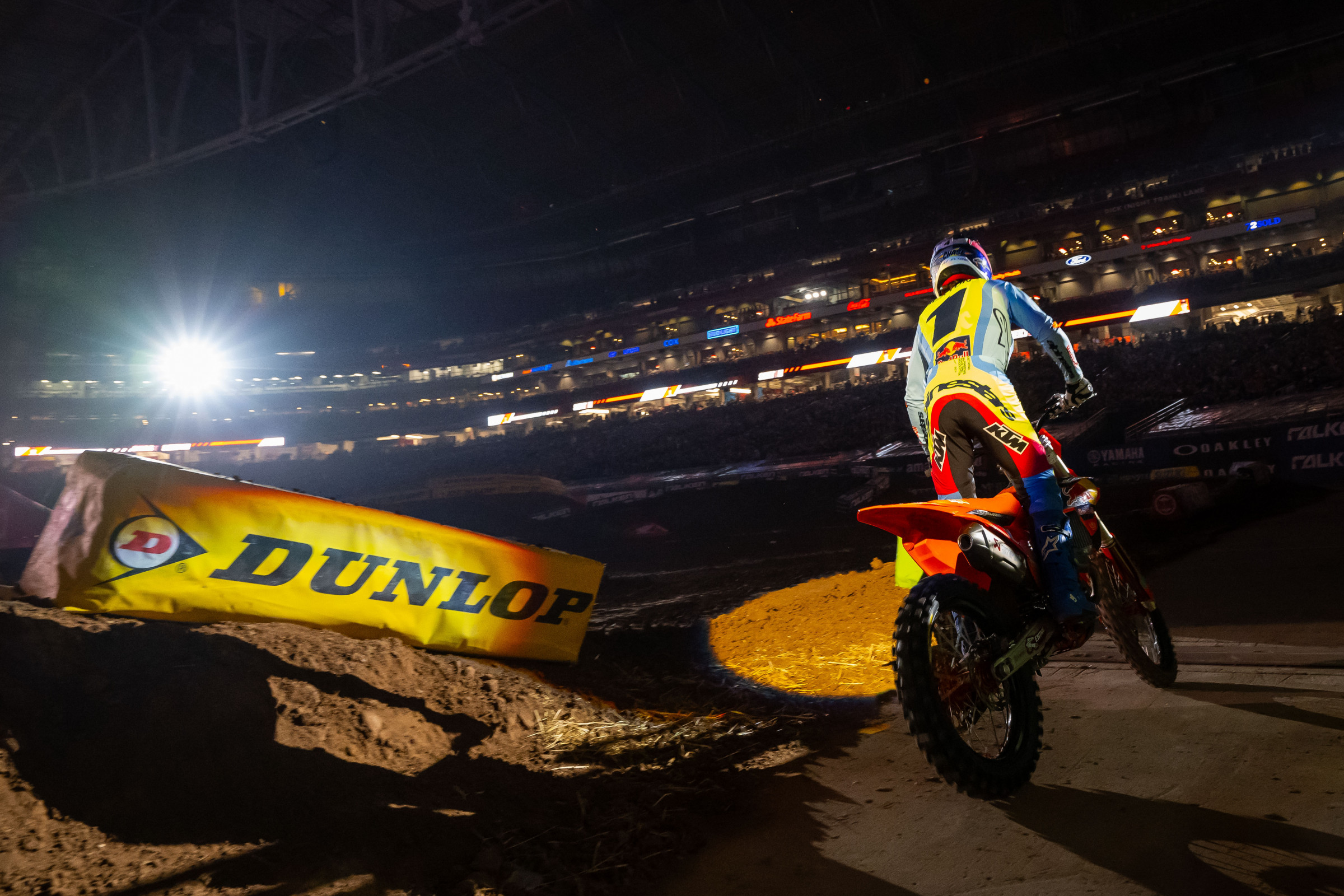In this vibrant night scene set in a circular arena, an illuminated motocross race unfolds under a dark sky obscured by city lights. The image centers on a motocross participant riding an orange motorcycle positioned to the right side, possibly preparing to make a turn. This rider, identifiable by the number 1 on their back, stands upright on their bike, dressed in a colorful suit of yellow, blue, and orange, complete with a helmet. The ground beneath is rugged, composed of dirt and rocks, typical for such events. The grandstands curve along the image’s periphery, filled with spectators and adorned with a variety of electronic banners in reds, blues, and yellows showcasing various sponsors. Notably, a prominent yellow 3D Dunlop banner with black lettering is visible on the left corner. The entire scene is brightly illuminated by a significant light source from the left, enhancing the vibrant atmosphere of the race.